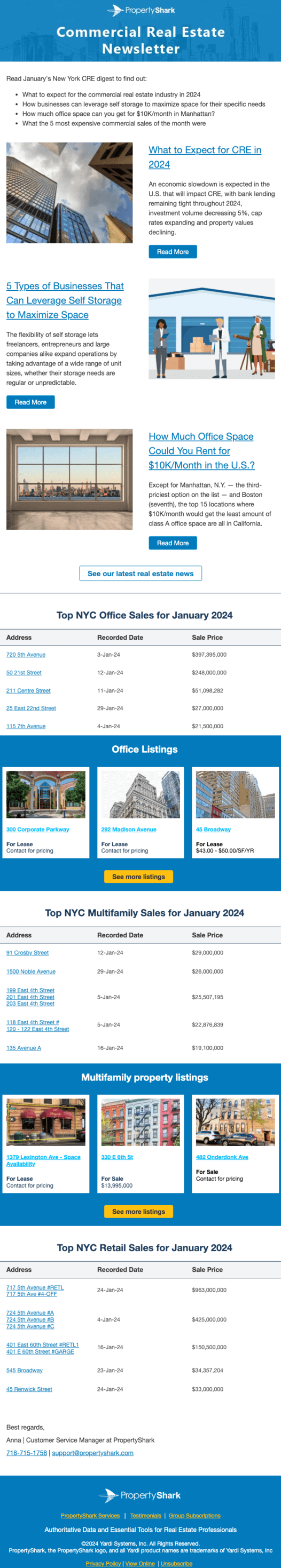The image is a detailed screenshot of a comprehensive infographic titled "Commercial Real Estate Newsletter." At the very top, an illustration depicts three individuals standing outside a building, setting the thematic tone. Just below this, the infographic is divided into multiple sections, each characterized by its distinct content and color scheme.

The first notable section, distinguished by a blue rectangular background, is labeled "Office Listings." Within this section, there are three photographs of different office buildings, each accompanied by pertinent descriptive text. A prominent yellow button is centrally placed within this area.

Moving further down, the next significant section, also with a blue background, is titled "Multifamily Property Listings." Similar to the previous section, it features three sub-sections, each displaying an exterior photograph of multifamily properties.

Nestled between these blue-background sections, there is another segment titled "Top NYC Multifamily Trends for January 2024," providing insights specific to the multifamily real estate market in New York City.

Finally, at the bottom of the infographic, another detailed segment is labeled "Top NYC Retail Sales for January 2024," likely summarizing notable transactions and trends within the NYC retail property market.

This vividly structured infographic offers a visually engaging and information-rich overview of the commercial real estate landscape, highlighting key listings and market trends for January 2024.